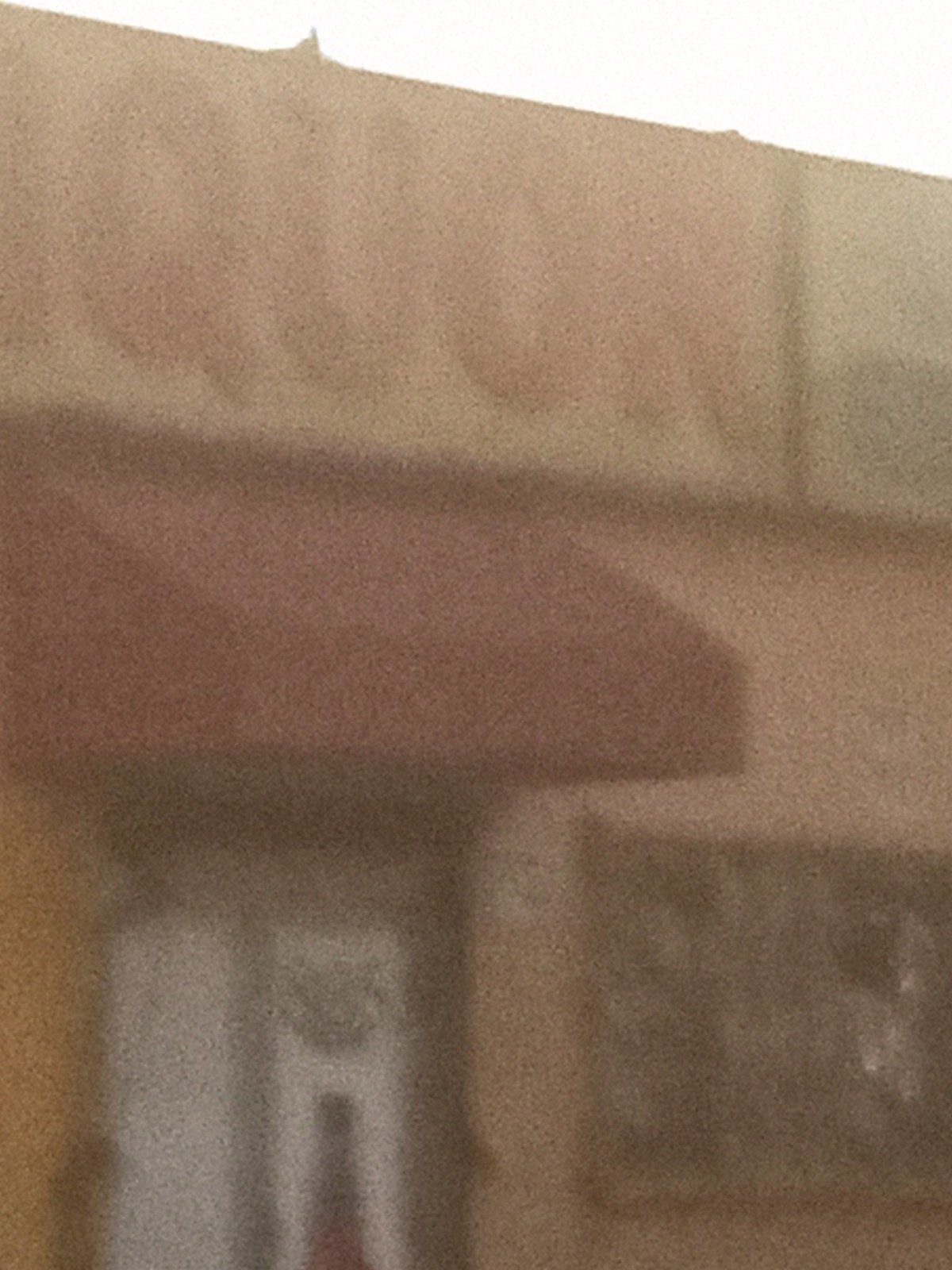The image depicts an extremely blurry and grainy storefront, bathed in warm, orange-yellow hues, with noticeable sunlight streaming in from above. The sign at the top of the building, though difficult to read, appears to contain the letters "I-Q-U-O-R" or "Q-U-O-R" in faint red against a whitish-pink background. Below the partially legible sign, a red or reddish-brown awning extends over a white door, which seems to feature black detailing, though it is also heavily blurred. Flanking the door is a blackened window that might be adorned with wrought iron. The overall structure of the building appears to be constructed of brown or red brick. Despite the significant graininess and out-of-focus elements, these details emerge from a thoroughly overexposed photograph.